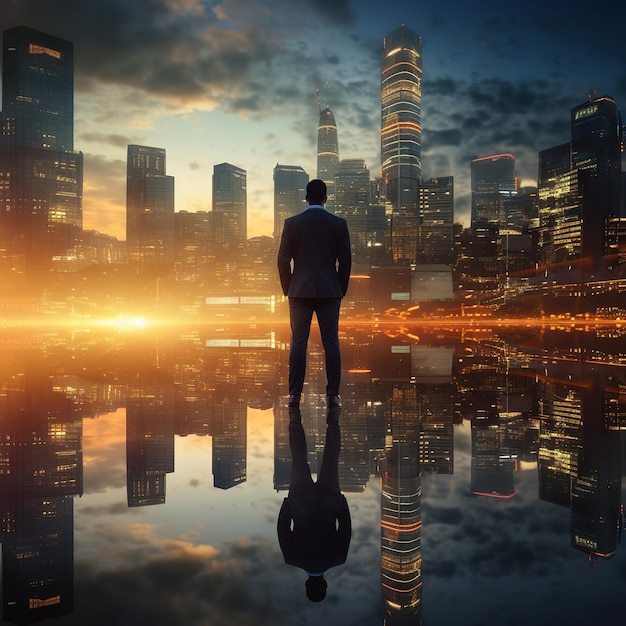In this evocative photograph titled "Contemplation," a tall businessman stands with his hands in his pockets, facing away from the viewer. He is positioned in the foreground, seemingly mesmerized by the sprawling cityscape before him. The city, bustling with towering skyscrapers, is vividly alive with a mix of glowing orange, yellow, and blue lights emanating from various windows and floors, creating a dynamic contrast against the darkening sky. The scene captures the cusp of nightfall, with a gradient sky transitioning from a lingering light blue to a deep, enveloping darker hue. Soft clouds still reflect the remnants of the setting sun, adding texture to the celestial canvas above.

The man stands on what appears to be a glass floor or a still body of water, mirroring the entire skyline and giving the illusion of an endless cityscape stretching beneath him. This reflective surface doubles the visual impact of the illuminated buildings and the twilight sky, enriching the overall composition. His clean-cut appearance, defined by a dark suit and a hint of a light blue shirt collar, contributes to the scene's sense of quiet admiration and introspection. Although his emotions remain hidden from view, his stance and the tranquil environment suggest a moment of serene contemplation, perfectly encapsulating the mood of the image.